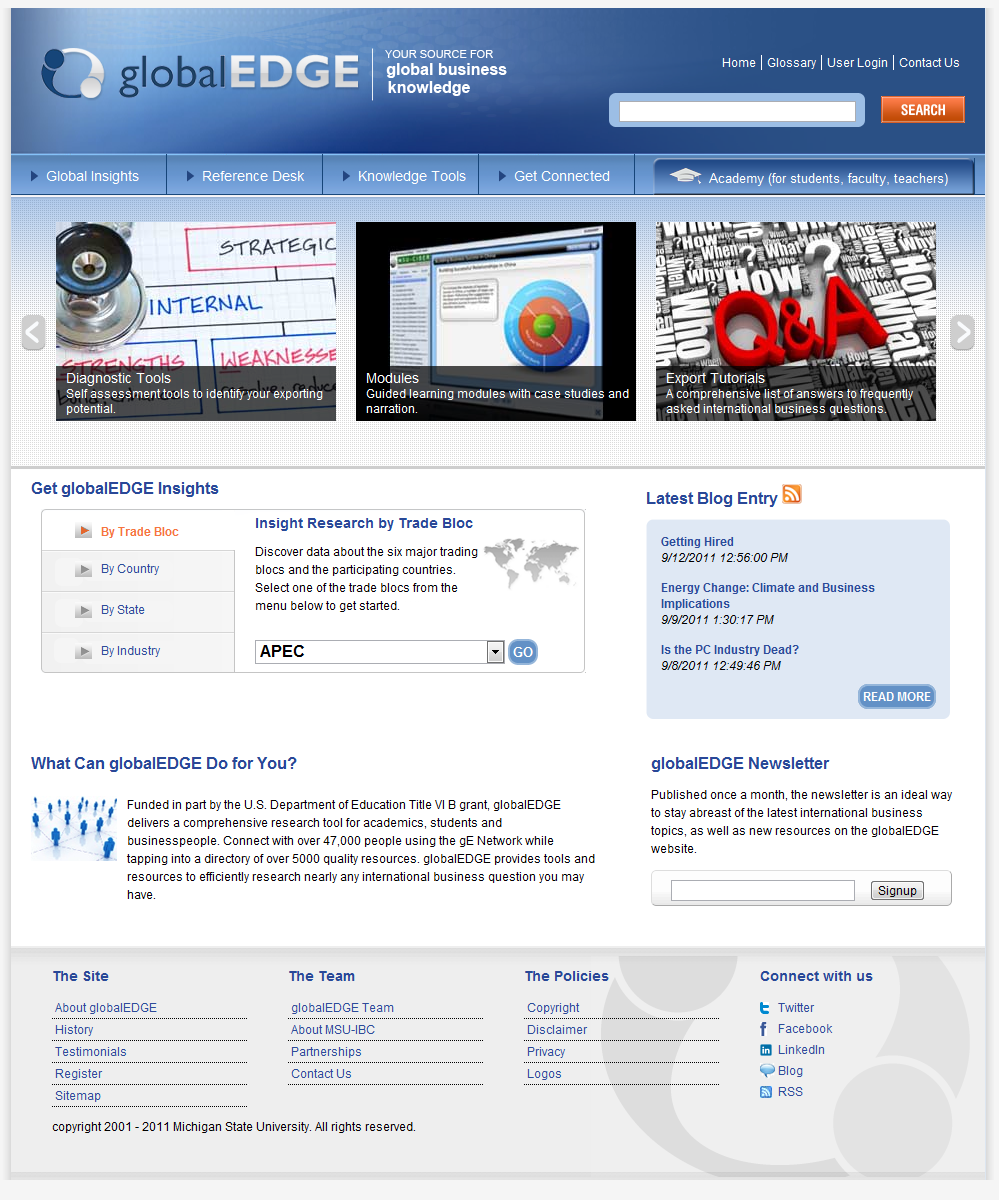In the upper left corner of the image, the logo reads "Global Edge," with 'Global' rendered in black or dark blue, and 'Edge' in bolded, white, capital letters. Adjacent to the logo, the tagline "Your Source for Global Business Knowledge" is displayed. On the right side of the header, navigation options including 'Home,' 'Glossary,' 'User Login,' and 'Contact Us' are listed, followed by a white search bar bordered in light blue, with a red 'Search' button featuring white text.

Beneath the header lies a row of navigation tabs: 'Global Insights,' 'Reference Desk,' 'Knowledge Tools,' 'Get Connected,' and 'Academy' (for students, faculty, and teachers). Below these tabs are three aligned images, each with descriptive text. The first image, on the left, promotes "Self-Assessment Tools to Identify Your Exporting Potential". The middle image advertises "Modules: Guiding Learning Modules with Case Studies and Narration". The third image highlights "Q&A Export Tutorials: A Comprehensive List of Frequently Asked International Business Questions".

Towards the bottom left of the image, a section titled "Get Global Edge Insights by Trade Block" provides research by trade block, country, state, and industry.